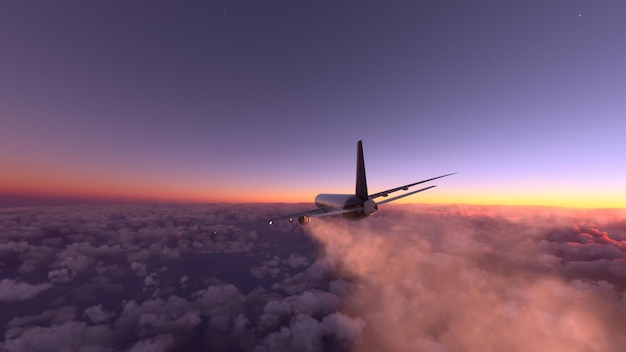This aerial photograph captures a detailed scene of a commercial airliner in flight during what appears to be sunset or sunrise. The aircraft, likely featuring four engines with visible exhaust trails, is primarily white with a possible blue tint and a black tail fin. The plane, slightly tilted, is framed in the right third middle of the image, flying across a breathtaking horizon bathed in shades of orange, pink, purple, and red. Below the horizon lies a sparse cloud layer, while above, the atmosphere presents a gradient from deep blue to a lighter blue, with at least one star visible in the top right corner. The composition, with the plane hovering above the scattered clouds, evokes a sense of tranquility and could easily serve as an advertisement or postcard.